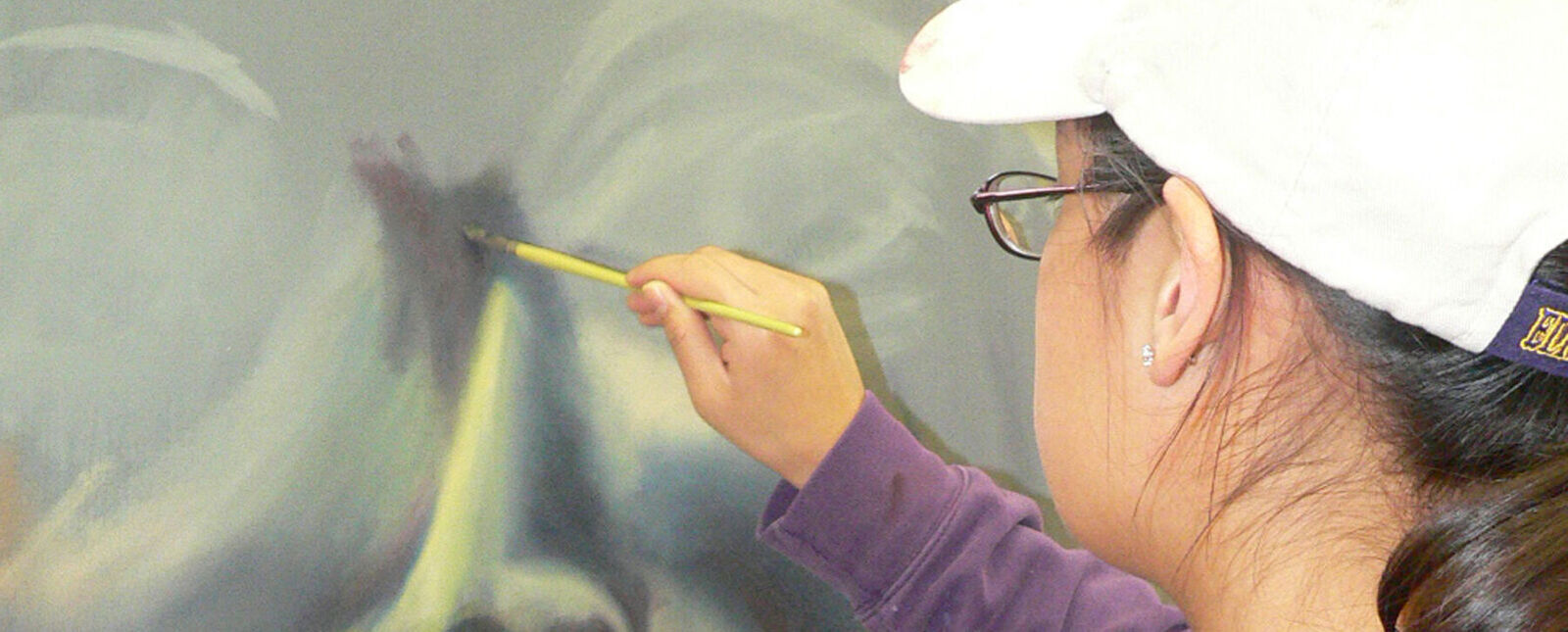The color photograph, staged and horizontal, shows a woman painting on a canvas. In the upper right corner, her white baseball-style cap fades into the whiteness, blending seamlessly with the screen's edge. The woman, who is likely of Caucasian or Hispanic descent, has brown skin and brown hair tucked under the cap. She wears black-rimmed glasses, with a diamond earring visible. The focus is on the left side of her head, showing her left ear and the left lens of her glasses. Her right arm, dressed in a long-sleeved purple shirt, holds a yellow paintbrush as she meticulously applies dark gray paint to a canvas already featuring lighter gray tones. The painting appears to depict a large face, with dark gray paint accentuating areas between light gray circles resembling eyes and a subtle yellow-tinted strip hinting at a nose. The image further reveals the faint outlines of eyebrows and eyes, with shading that suggests cheekbones, adding depth and dimension to the emerging portrait.